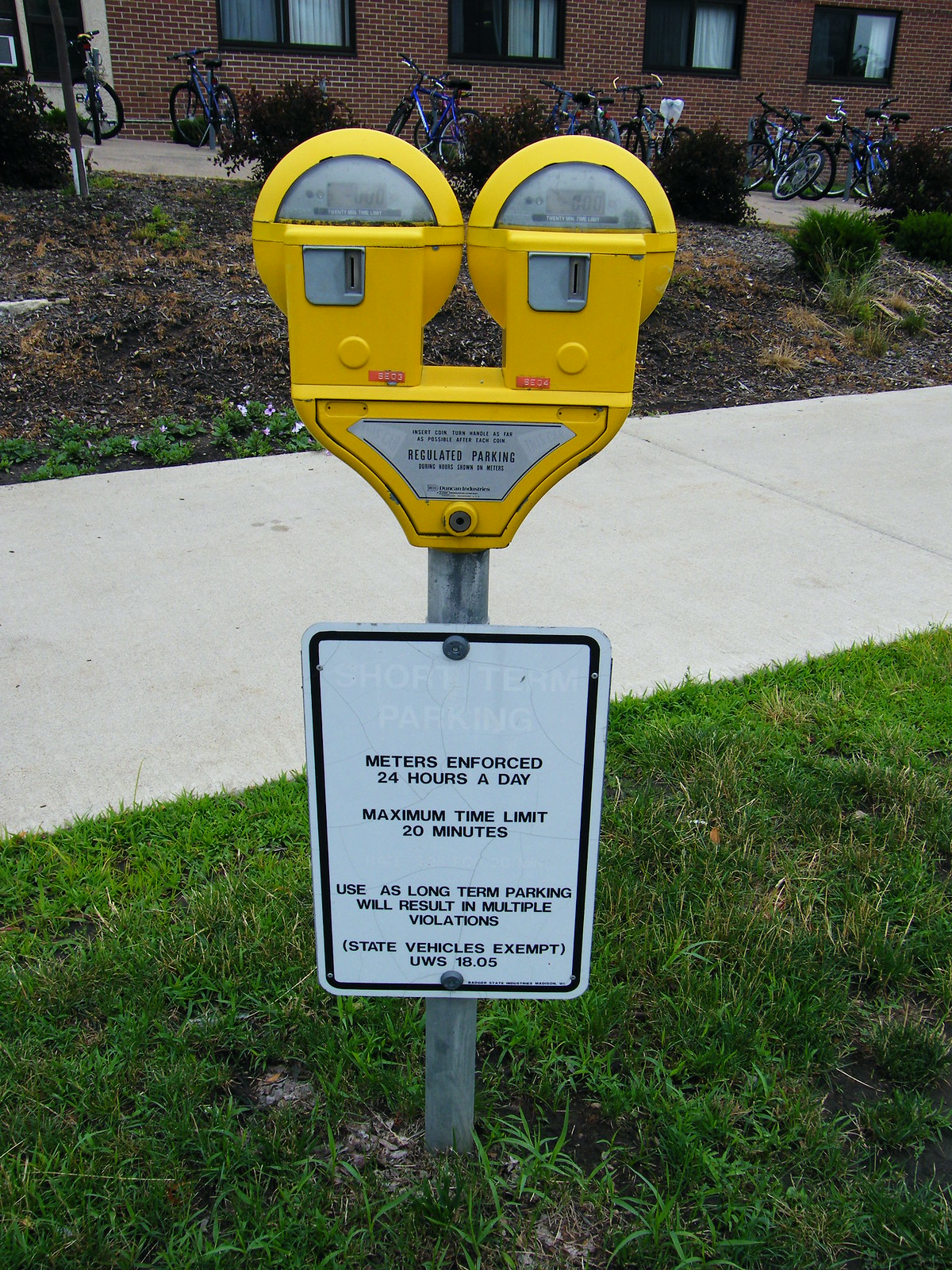This detailed color photograph captures a yellow, dual-head parking meter with a steel silver pole situated in a small patch of green grass. The meter features coin inserts on both its left and right sides and displays a digital readout indicating the remaining parking time. Riveted to the pole is a white sign with black lettering, reading: "Short-term parking meters enforced 24 hours a day, maximum time limit 20 minutes. Use as long-term parking will result in multiple violations. State vehicles exempt." In the background, behind a white concrete sidewalk, lies a dirt patch sparsely dotted with green shrubs. Beyond this, a reddish-brown brick building with dark-trimmed windows and curtains stands prominently, featuring a doorway and several windows. Approximately seven blue bicycles are neatly parked in a bike rack against the brick wall. The focus and sharpness of the image suggest it was taken with a high-quality camera.